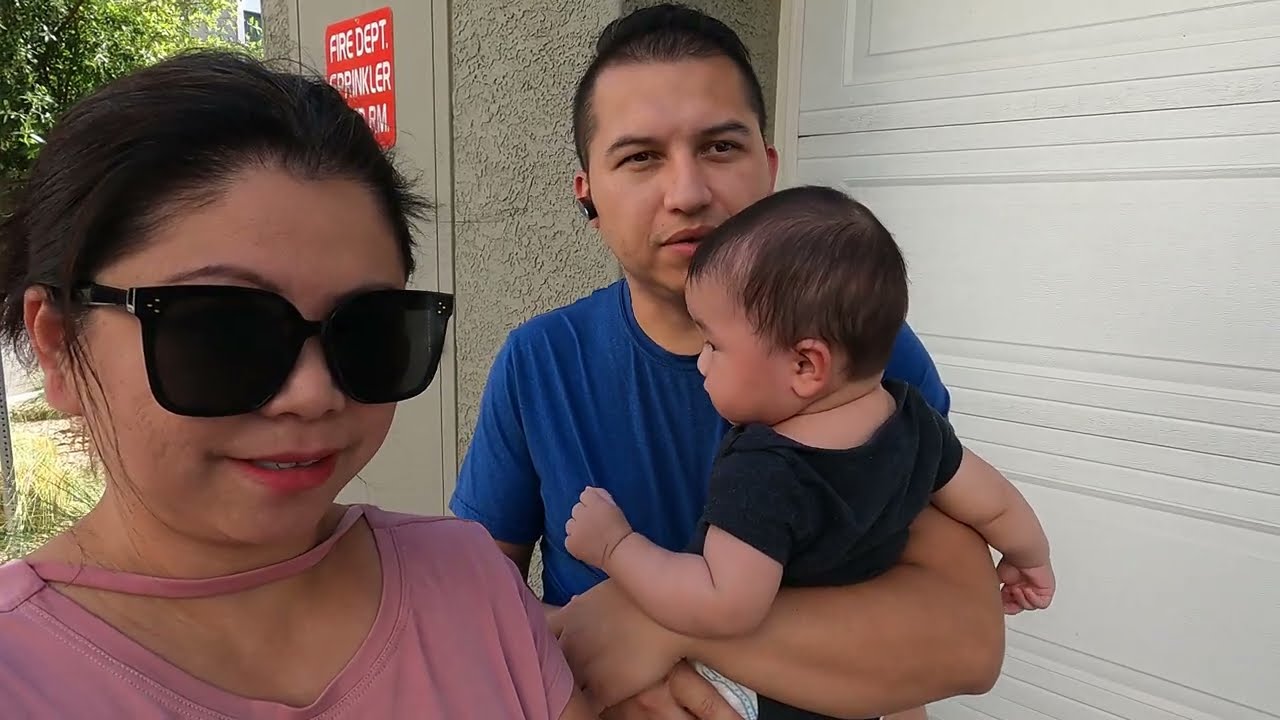A family of three stands together in an outdoor setting. The father, at the center of the photo, wears a dark navy blue shirt and has a wireless earbud in his right ear. He cradles a baby in both arms, who wears a black shirt and has brown hair. The father is looking slightly to the right, while the baby gazes off to the left. To their left stands the mother, smiling widely. She is dressed in a light pink shirt with a V-shaped neckline and has her hair tied back in a ponytail. She accessorizes with large black sunglasses. Behind them, a white garage door is visible, and to the left of it a door with a sign that reads "Fire Department Sprinkler Alarm." In the background, there are green trees and grass, contributing to the outdoor atmosphere.